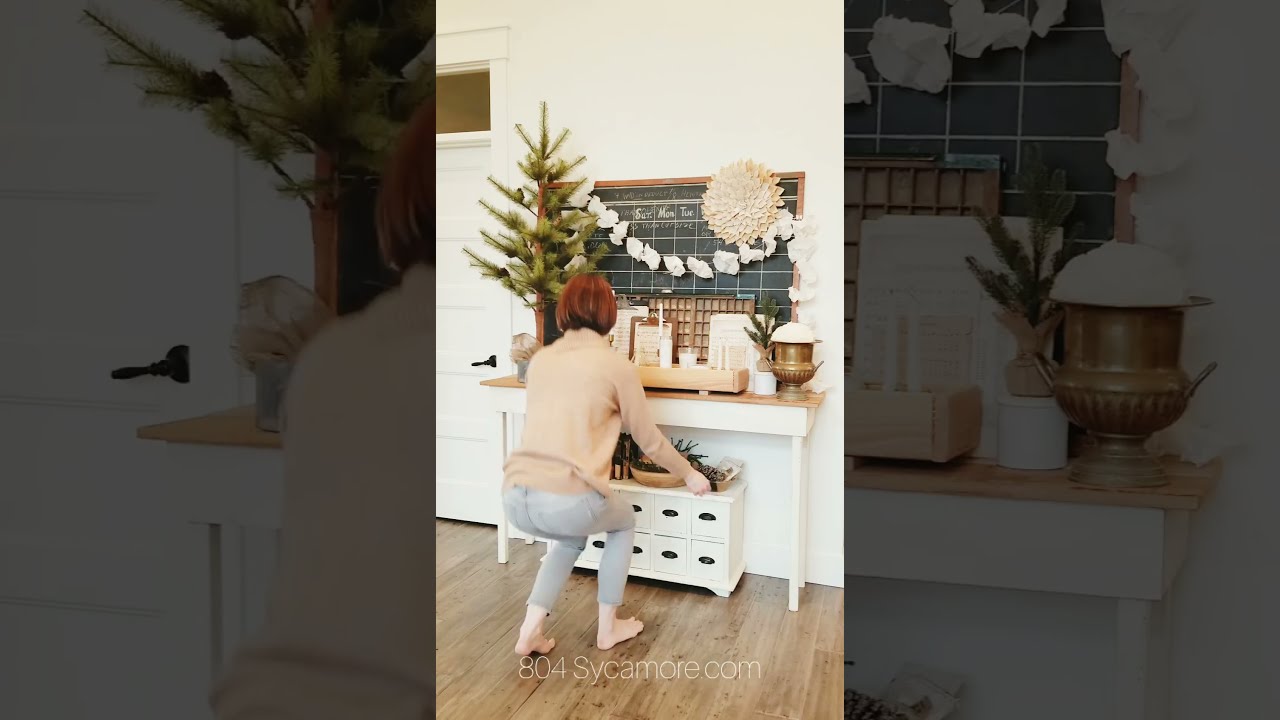The image features a central, tall rectangular photograph framed by wide black borders on the left and right sides. The scene depicts a light, homey, indoor setting. A barefoot woman with short red hair, wearing gray pants and a beige turtleneck sweater, is captured mid-step, walking to the right. Her left heel is lifted as she moves forward. She stands on a light brown wooden floor, adding warmth to the environment. In the background, there's a crisp white wall with a white door slightly visible on the left. Directly behind her, a narrow table with a light brown wooden surface holds a variety of homey, earthy decorations, including a small Christmas tree adorned with a white garland, a wooden box, a bowl, a candle, and a chalkboard calendar. Below the table, a small chest of drawers adds to the room's cozy, organized feel. At the bottom of the image, in white font, the text "804sycamore.com" suggests an advertisement or possibly a promotional website video. The balanced composition and detailed setting evoke a sense of warmth and home comfort.